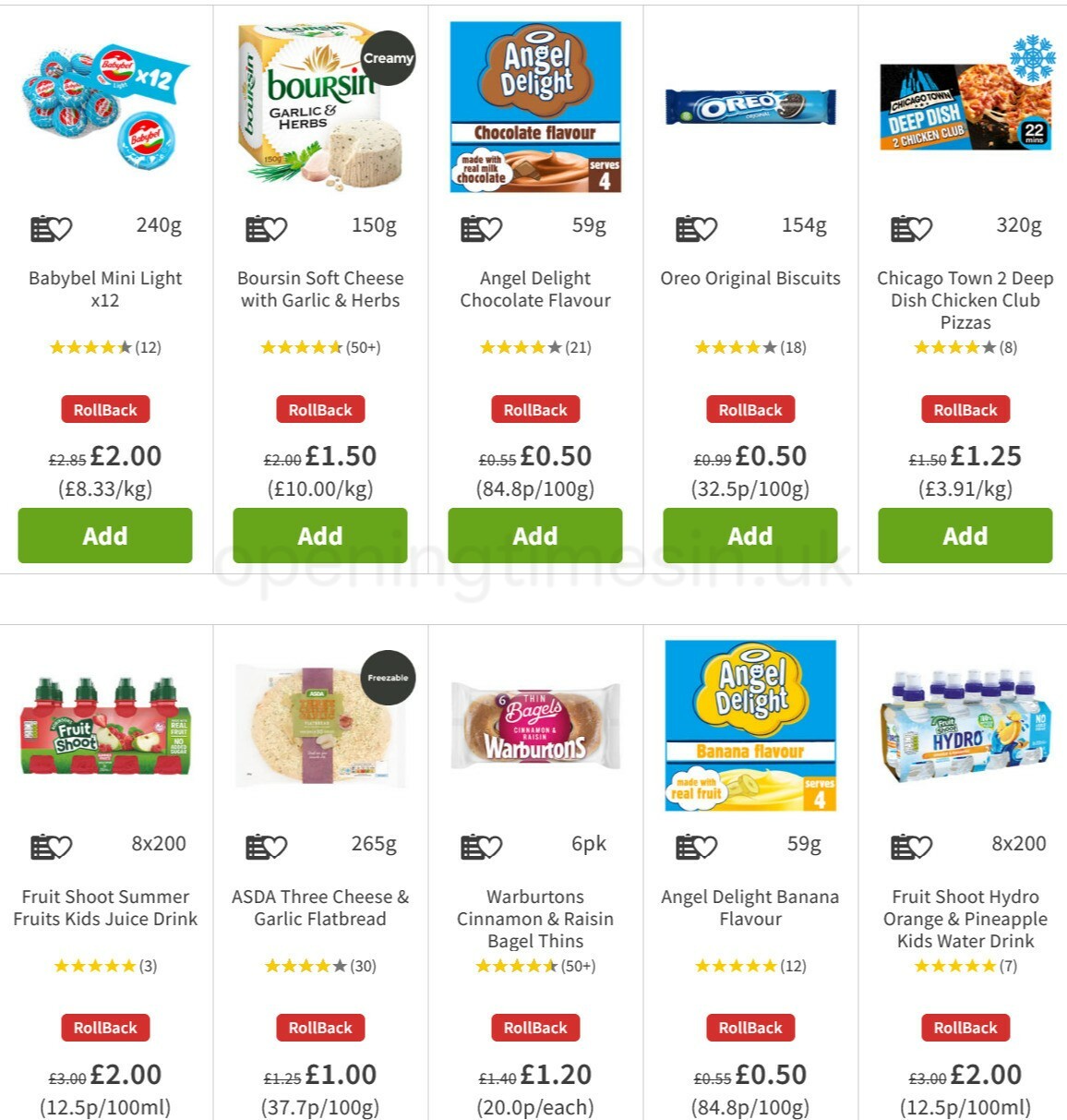This screenshot showcases a grocery shopping website's interface, organized into two distinct rows each featuring five product categories. 

**Top Row:**

1. **Mini Light Cheese**  
    - Features an image, detailed description, and user rating (yellow stars). 
    - A red "Rollback" button indicates a price reduction, showing the original price struck through and the current price in pounds.
    - A green "Add" button with white text for adding the item to the shopping cart.

2. **Garlic and Herb Cheese**  
    - Includes product image, description, and yellow star rating.
    - Presence of a red rollback, discounted price marked, and actual price in pounds.
    - Green "Add" button for easy inclusion in the shopping cart.

3. **Chocolate Flavour Pudding**  
    - Displays product image, brief description, and rating stars.
    - Red rollback button shows a discounted rate; original and actual price in pounds are shown.
    - Green "Add" button to add the item to the cart.

4. **Oreos**  
    - Image and brief description provided with user rating stars.
    - Red rollback for discount indication; crossed-out original price and current price in pounds shown.
    - Green "Add" button for adding the item.

5. **Deep Dish Pizza**  
    - Contains product image, description, and star ratings.
    - Red rollback button reflects a price cut with original and current price in pounds.
    - Green "Add" button for easy shopping.

**Bottom Row:**

1. **Fruit Shoot**  
    - Product image, description, and star ratings are presented.
    - Red rollback button shows the discount; original price crossed out and current price in pounds.
    - Green "Add" button to add to the shopping cart.

2. **3 Cheese Flatbread**  
    - Features an image, brief description, and star rating.
    - Price reduction indicated by the rollback button; original and actual price shown in pounds.
    - Green "Add" button available for adding the item.

3. **Warburton's Bagel Thins**  
    - Shows product image, description, and user rating stars.
    - Red rollback button with discounted price marked; original price struck through.
    - Green "Add" button for adding the item.

4. **Angel Delight Banana Flavour**  
    - Displays product image, brief description, and star ratings.
    - Rollback button indicates a reduced price; original price crossed out and current price in pounds.
    - Green "Add" button for easy addition to the cart.

5. **8 Pack of Water**  
    - Image, description, and user star ratings are indicated.
    - Red rollback button shows price cut, with the original price struck through and the actual price in pounds.
    - Green "Add" button to add the item.

Additionally, below each row, there is an option to add items to your shopping list and see descriptions with detailed ratings. The rating system largely shows five stars with the exception of one item in the second row rated four out of five. Prices are specified per unit of measurement for precision.